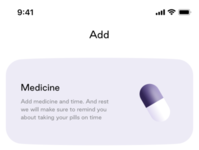The image is a screenshot from a cell phone, as evidenced by the time displayed in the upper left corner, which reads 9:41. The status bar also shows the strength of the cellular signal and the battery life. The main content of the screen is an app interface that appears to be a medication reminder. At the top, there is a label that says "Add Medicine," followed by an icon of a purple and white capsule pill. Below this icon, there are three lines of text that are blurry and difficult to read, but it suggests instructions or details related to adding medication. The app likely serves as a reminder tool to help the user keep track of their medication schedule, possibly offering features to alert the user when to take their pills or when they are running low. The interface indicates functionality for adding specific medications, ensuring the user takes certain pills at designated times.